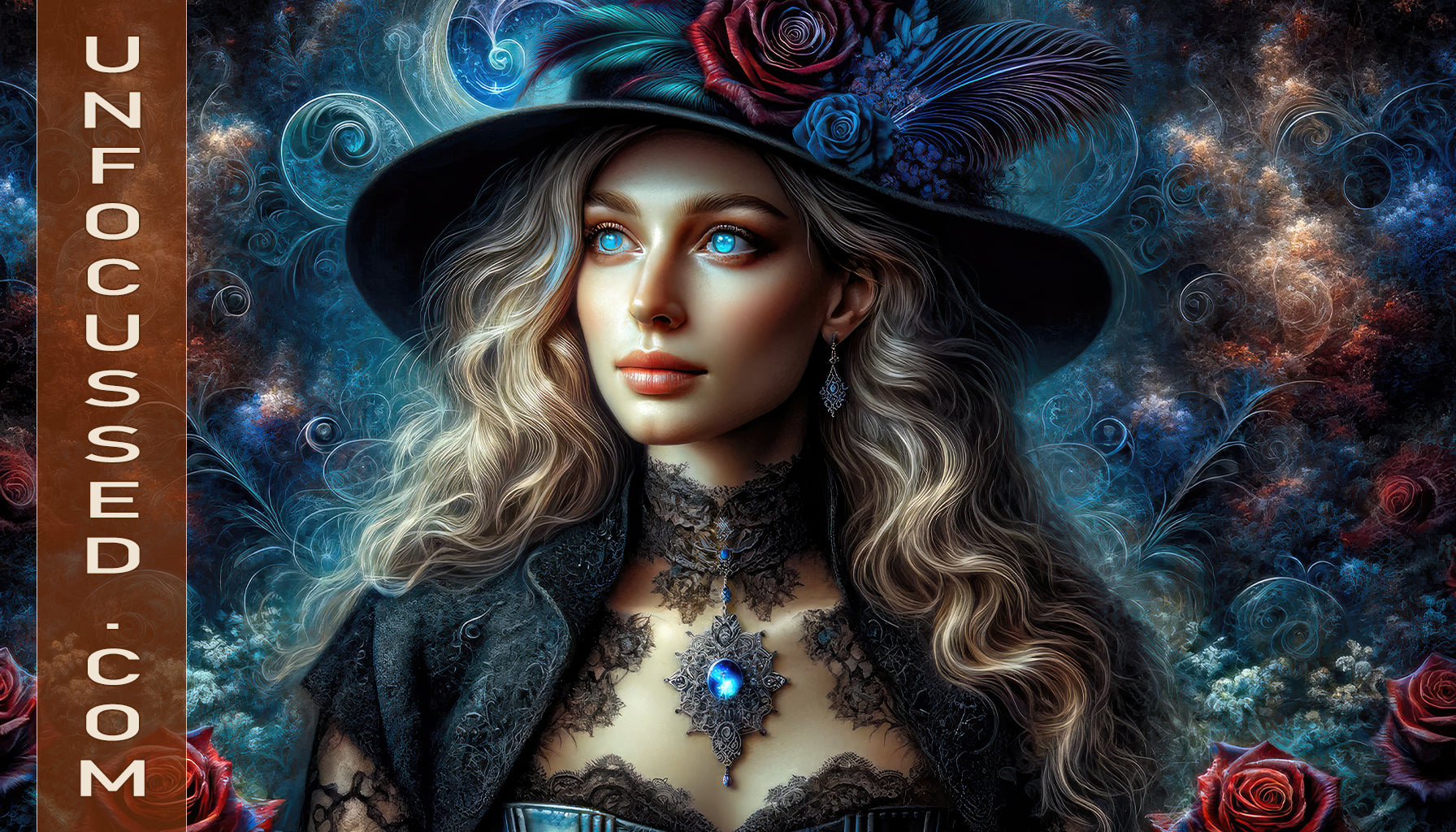The image is a highly detailed digital artwork or AI-generated illustration of a woman's face and upper torso. The background features an intricate, foggy blue pattern with abstract curves, roses, and bird feathers. The woman, depicted from her chest upwards, has bright blue eyes, slightly blushed cheeks, and pink lips. Her long, blonde curls cascade past her shoulders. Adorning her head is a large, dark green hat embellished with flowers, including a dark purple peacock feather and a dark red rose. She wears a black corset with frilled top, under a crop top black coat, and a thick, frilly black choker around her neck. From the choker hangs a silver, diamond-shaped pendant with a prominent round blue stone. A brown, semi-transparent banner runs vertically along the right side of the image, with white text reading "unfocussed.com" (spelled as U-N-F-O-C-U-S-S-E-D period C-O-M).